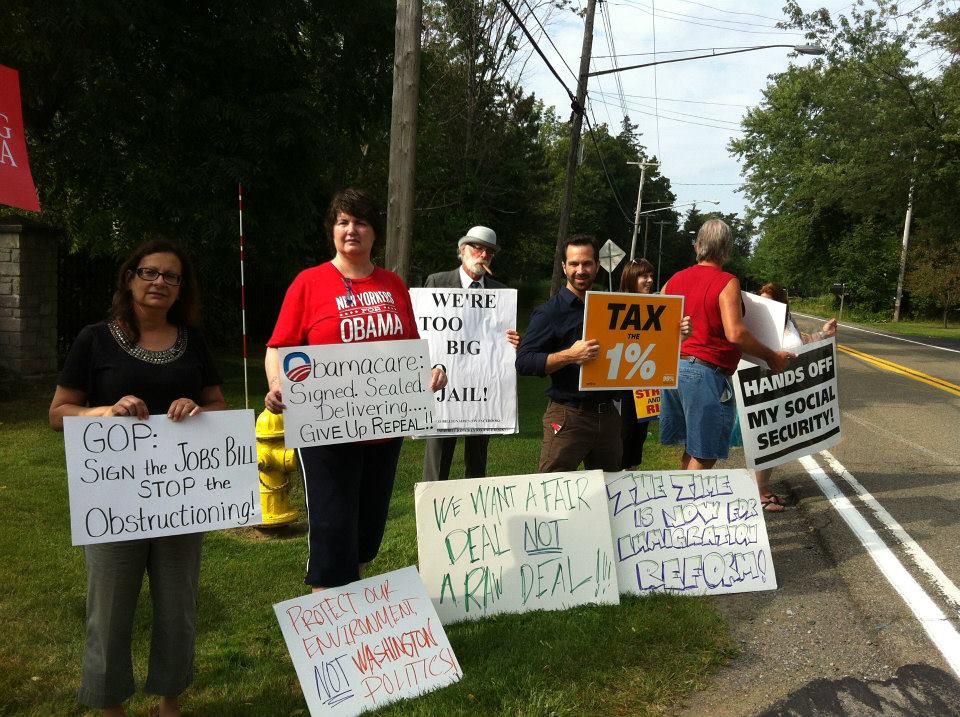In this vibrant daytime outdoor country street scene, a small group of casually dressed individuals is shown standing on the grass beside an asphalt road, holding various political signs. The road, marked by white outer lines and a central yellow line, is bordered by wooden telephone poles and flanked by trees on both sides. A yellow fire hydrant, featuring a red and white snow stick, is visible in the background.

On the left of the image, a woman wearing glasses, a dark top, and grey pants holds a white sign that reads, "GOP, sign the jobs bill, stop the obstructioning." To her right, another woman in a red short-sleeved top and black pants holds a sign about Obamacare saying, "Obamacare, signed, sealed, delivered. Give up repeal," and another one at her feet stating, "Protect our environment, not Washington politics." Next is a man in the background with a white derby hat, a large white beard, and a cigar in his mouth, dressed in a grey suit and a white collared shirt with a tie. His sign proclaims, "We're too big to jail," with another at his feet reading, "We want a fair deal, not a raw deal."

Continuing to the right, another man wearing a dark blue shirt and brown pants shows a sign that says, "Tax the 1%," with an additional sign below him stating, "The time is now for immigration reform." Further to the right, a man in a sleeveless red shirt and blue shorts holds a sign that demands, "Hands off my social security." Another unidentified individual with their back to the camera, also dressed in a red top and blue pants, is partially visible holding a similar sign. The scene captures a clear, summer-like day filled with political activism and a call for legislative action across various issues.